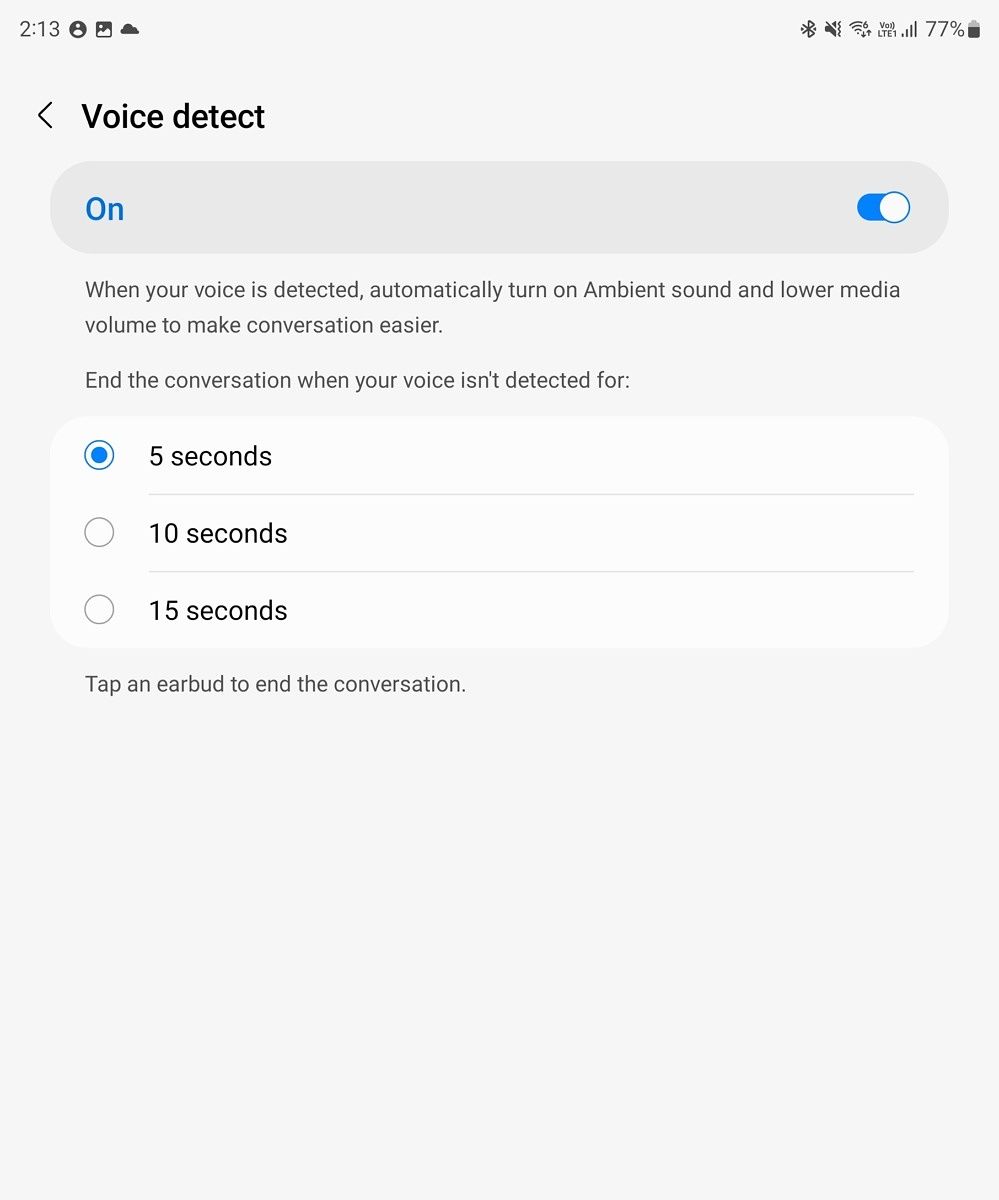The image depicts a screenshot from a website featuring a settings interface for a cell phone. At the top of the interface, there are menu selections with "213" on the left side and a "Volume Off" icon, indicating mute mode, on the right. The battery level is displayed at 77% with a Bluetooth indicator next to it.

The main section of the screen describes a feature titled "Voice Detect," which is currently toggled on, denoted by a blue switch on the right side. This feature enables the phone to detect when the user's voice is recognized, automatically turning on ambient sound and lowering media volume to facilitate easier conversation. The toggle switch is highlighted in blue.

Below this description, there’s an option to set the duration for which the ambient sound feature should remain active after detecting the user's voice. The options are listed as five seconds, ten seconds, and fifteen seconds. Each option is preceded by a circle, with the circle next to 'five seconds' selected and filled in blue.

The background of the settings interface is gray, with black font used for the text. The selectable options (five seconds, ten seconds, fifteen seconds) are displayed on a white background and separated by thin gray lines. The toggle for turning on the "Voice Detect" feature, as well as the selected circle, are prominently marked in blue. The overall design utilizes horizontally elongated rectangles for all interactive fields, contributing to a clean and organized layout.